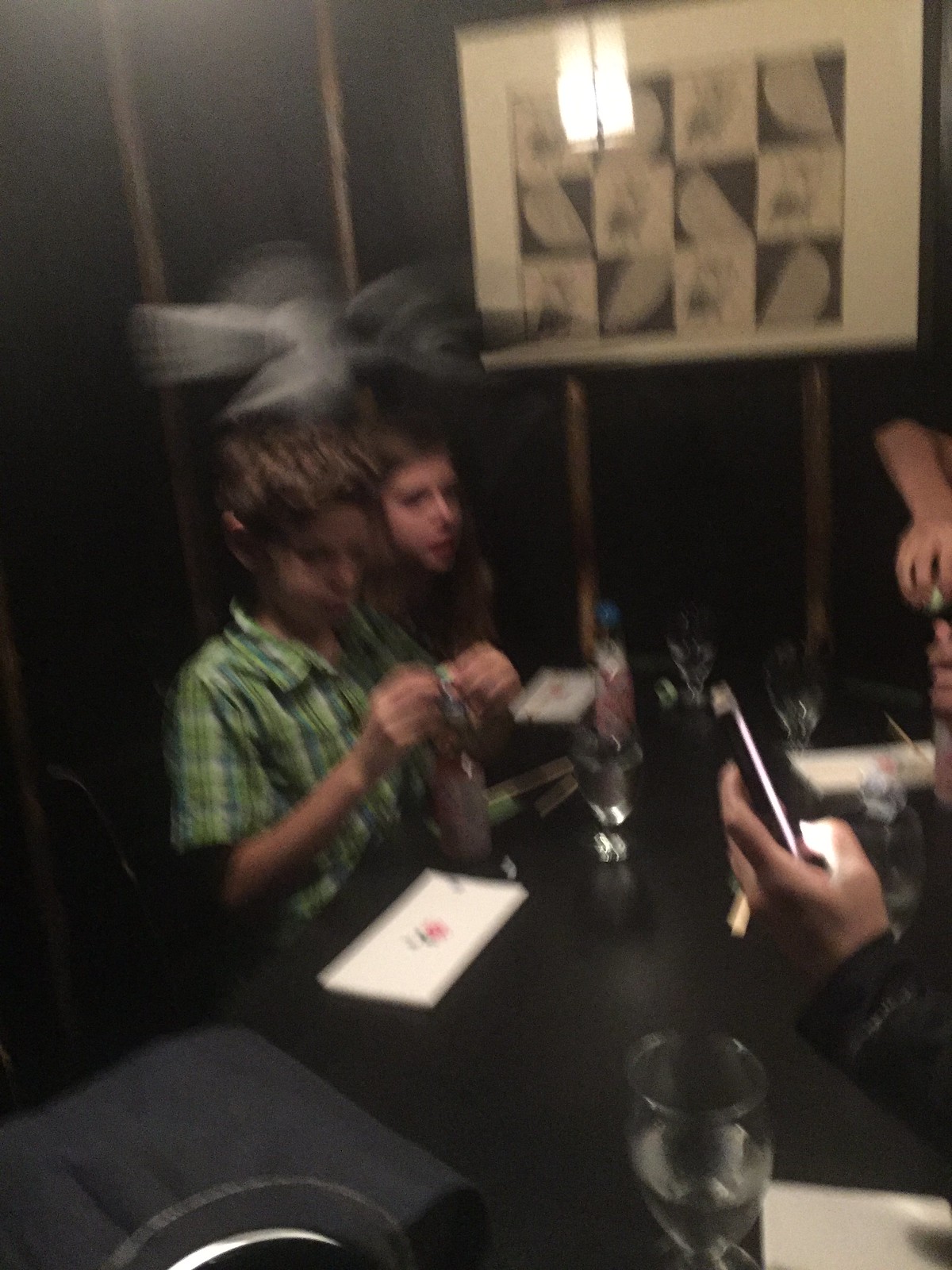In this photograph, a family is seated at a long black table, possibly in a restaurant booth. Prominently featured on the left side of the image are a young boy in a green plaid button-up shirt and a girl with brown hair. The girl appears slightly older than the boy, although her outfit is not visible. The children sit across from their parents, whose presence is only hinted at through partial views—such as a left hand typing on a smartphone and a right arm—indicating they are seated on the right side of the table. Scattered across the table are several items, including clear drinking glasses filled with water, a wine glass on the bottom right, napkins, chopsticks, and a large rectangular piece of paper near the boy. The boy seems to be adding something to his drink. Adorning the wall behind them, which is black with gold trim, is a large framed picture. The image conveys a lively, informal dining experience despite having some blurred elements.